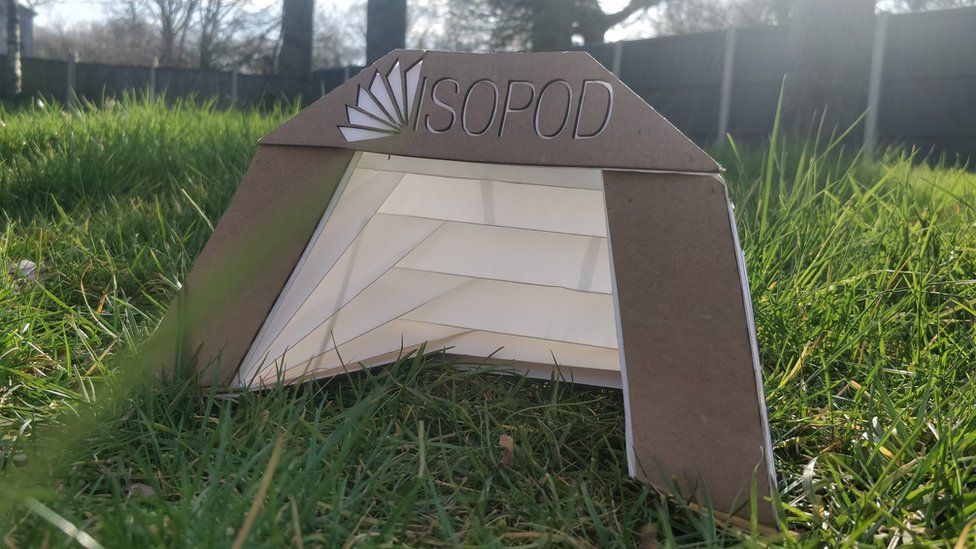In a sprawling, untamed backyard with ankle-length grass and a view of a large wooden fence and leafless tall trees under a daytime sky, there sits a peculiar rectangular structure on the ground, prominently featuring a tent-like design. This small structure, which has brown sides and a trapezoidal top, showcases a distinctive arrangement: its front is divided into three sections, each rendered in brown. The top section is shaped like a chimpanzee and bears the word "IZOPORT" in all caps, with a logo of six white triangles on its left side. Each side of the tent has a parallelogram-shaped area and features a triangle. The structure has a unique white accordion-fold design at the back, resembling vents, potentially indicating its function as a makeshift pet house. The wild, unkempt green grass and the gray fence with light-colored posts frame this curious object, contributing to the rustic outdoor setting.